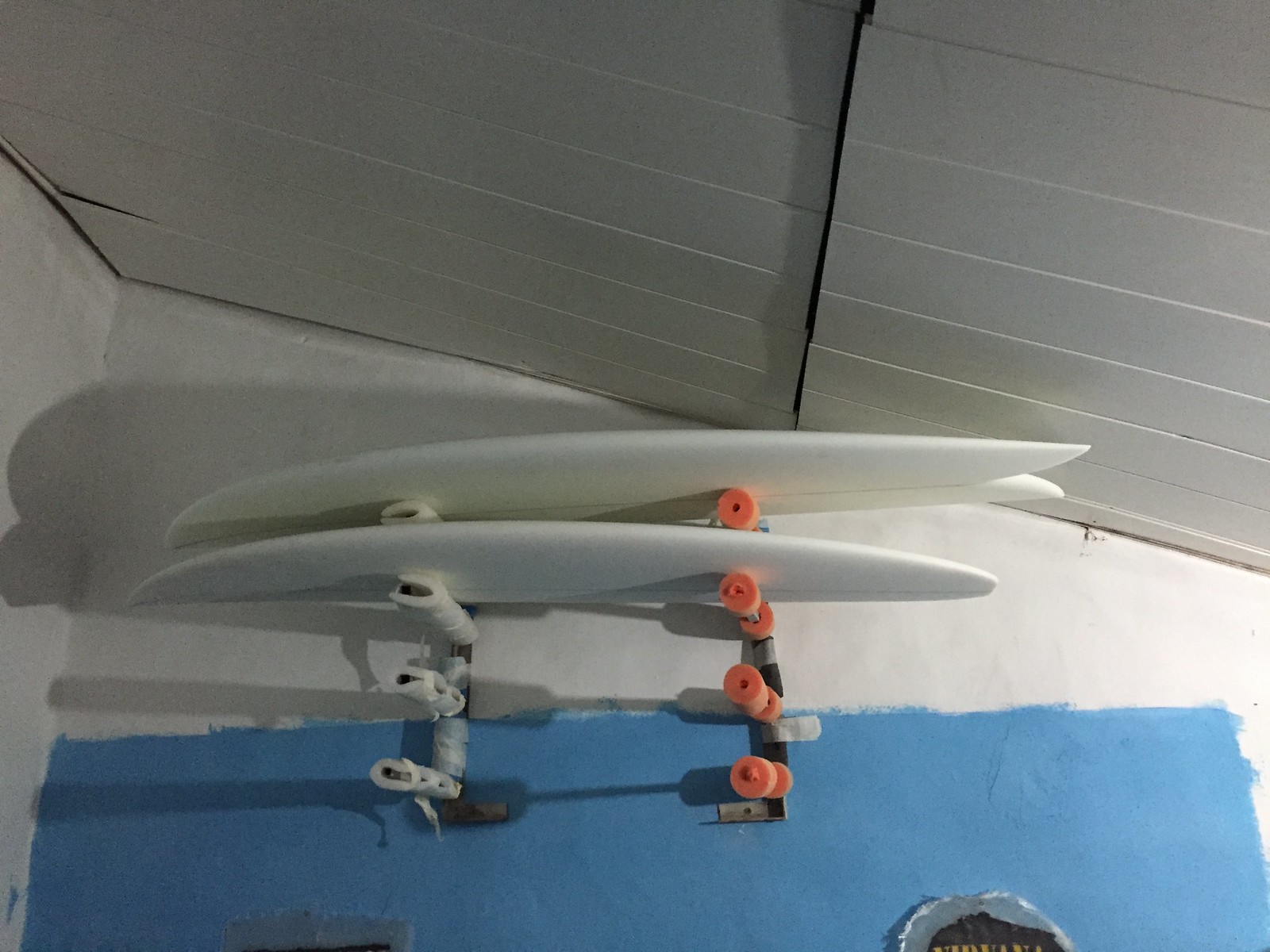This color photograph captures the interior of a room with a slanted white ceiling. The background features a gray wall segmented into two parts, with what looks like a crack on one of the siding planks on the left. Dominating the wall is a rack divided into two sections: the left segment adorned with white, peg-like items and the right hosting orange ones, resembling skateboard wheels. Perched horizontally on the top two spaces of this rack are two white items, appearing too short to be standard surfboards but shaped similarly. Below the rack, the wall transitions into a painted blue segment. Shadows of these objects are cast onto the wall, enhancing the detailed textures and contrasts in this thoughtfully composed scene.